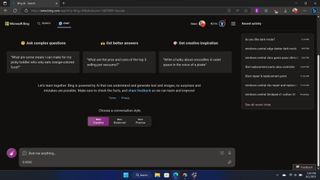The image is a small screenshot taken from the desktop of either a PC or a laptop, employing the Windows 11 operating system, as identified by the distinctive layout of the taskbar at the bottom. The screenshot captures a web browser window displaying a webpage characterized by a completely black background. The webpage features several gray boxes with white text, although the text is too small to be legible. Notable elements include two buttons illuminated in purple: one situated in the lower left corner, possibly a chat button, and another purple square above it. Adjacent to these purple elements are two black squares containing additional white text. Despite the text being unreadable, the overall layout suggests an interface with interactive elements and a dark-themed design.